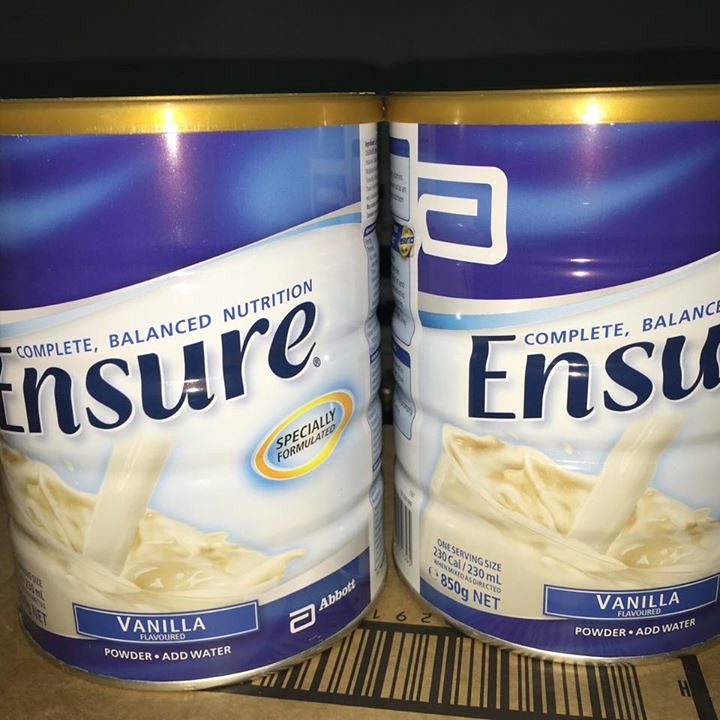The image depicts a pair of tin steel cans of Ensure Vanilla Flavored Powder with a focus on their detailed labeling and packaging, illuminated by a bright light that creates a stark contrast against a black void at the top. Both cans are lying on a flattened shipping carton with a large, visible UPC code in black. Each can features a prominently displayed blue label that highlights the "Ensure" brand logo, and above it, the text "Complete Balanced Nutrition." Below the brand name, a gold circle contains the words "Specially Formulated." An image of a creamy vanilla drink being poured into a glass graces the label, symbolizing the product inside. At the bottom of the label, a blue rectangle area showcases the text "Vanilla Flavored," and below it, the words "Powder. Add Water." The logos of the company, Abbott, are visible on both the label and the blue-colored plastic lid. The right can is slightly turned, revealing additional nutritional information, including "230 cals for 230 mls" for one serving size and a net weight of 850 grams. This meticulous arrangement captures the essence and branding of the product while providing a clear view of its packaging elements and nutritional claims.